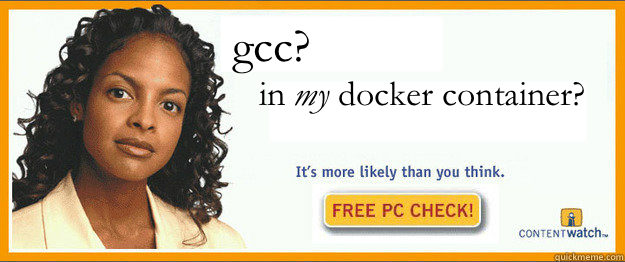A professionally dressed Black woman, wearing a cream-colored suit with her hair down, stands confidently. The text beside her reads, "GCC in my Docker container? It's more likely than you think. Free PC check, content watch." This modern twist is a clever homage to the classic internet meme that humorously warned, "porn on my computer? It’s more likely than you think." The meme, which dates back at least a decade, originally played off an advertisement. In this updated version, "GCC" refers to the GNU Compiler Collection for C in Linux, and "Docker container" refers to a standard unit of software that packages code and its dependencies, often used for developing and deploying applications.